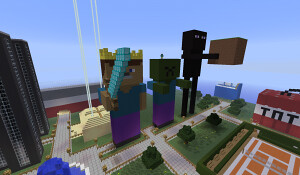A diminutive rectangular photograph depicts several Minecraft characters standing on a platform that resembles a walkway, with lush trees in the foreground. The central character, clad entirely in purple, brandishes a sword. Beside him, another character with darker skin also wears purple attire. Adjacent to them is an Enderman, a tall, completely black figure, holding a block. Scattered around are red and white TNT blocks, suggesting a potential explosive scene. The surroundings are adorned with greenery and an abundance of trees. On the left side of the image, an imposing structure resembling an office building, complete with numerous windows and an elevator system, stretches skyward. Additional orange and white blocks add vibrant accents to the scene. Overall, the image captures the essence of Minecraft, a game centered around constructing and exploring blocky worlds.